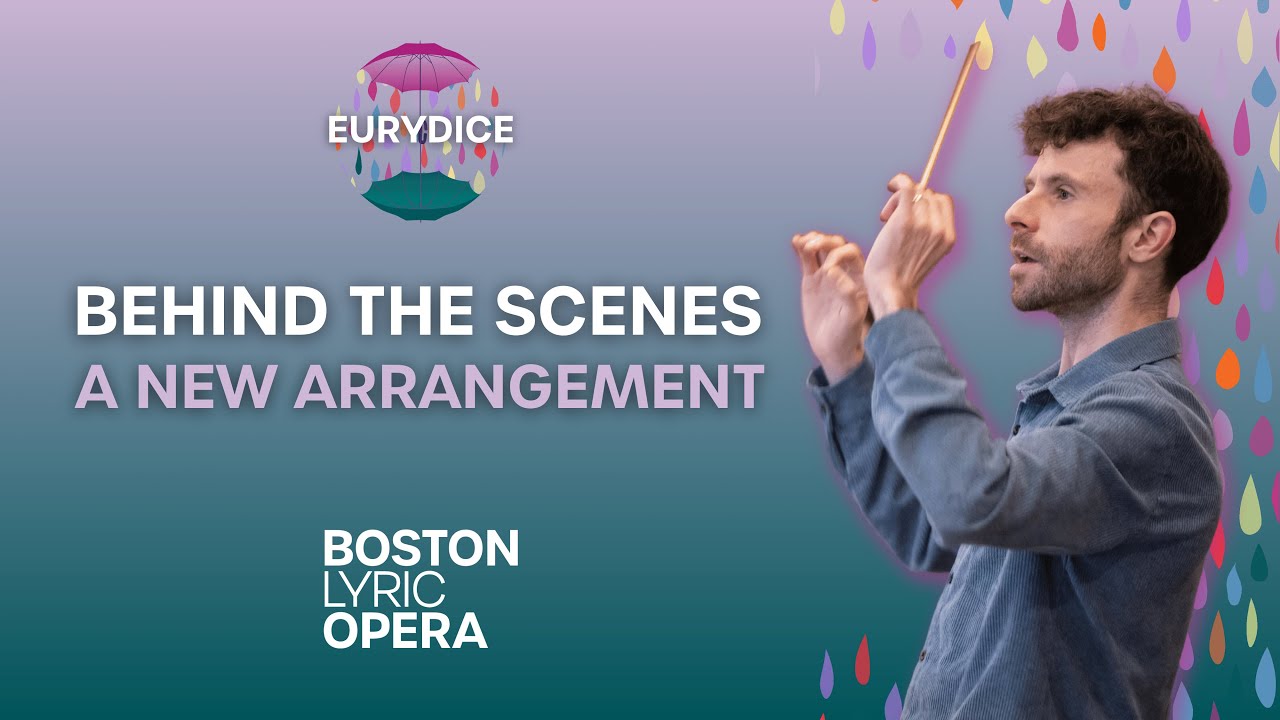The image appears to be an advertisement for the Boston Lyric Opera, featuring a comprehensive and colorful design. Centrally, the logo for "Eurydice" (spelled E-U-R-Y-D-I-C-E) is prominently displayed, featuring two umbrellas – one pink and one teal – mirroring each other with a cascade of colorful raindrops within the design. 

On the right side of the image stands a white male conductor, dressed in a regular button-up, long sleeve gray shirt. He has brown curly hair and a beard, and is holding a conductor's baton in his left hand, poised as if directing an orchestra. Surrounding him are vibrant raindrops in shades of orange, purple, yellow, and blue, creating a dynamic and visually engaging effect.

To the conductor’s left, the text "Behind the Scenes" is written in bold white letters, followed by "A New Arrangement" in lilac purple, and "Boston Lyric Opera" in bold white letters below. The background of the image features a striking gradient, starting with teal at the bottom and transitioning into lilac purple towards the top, adding to the overall aesthetic appeal of the advertisement.